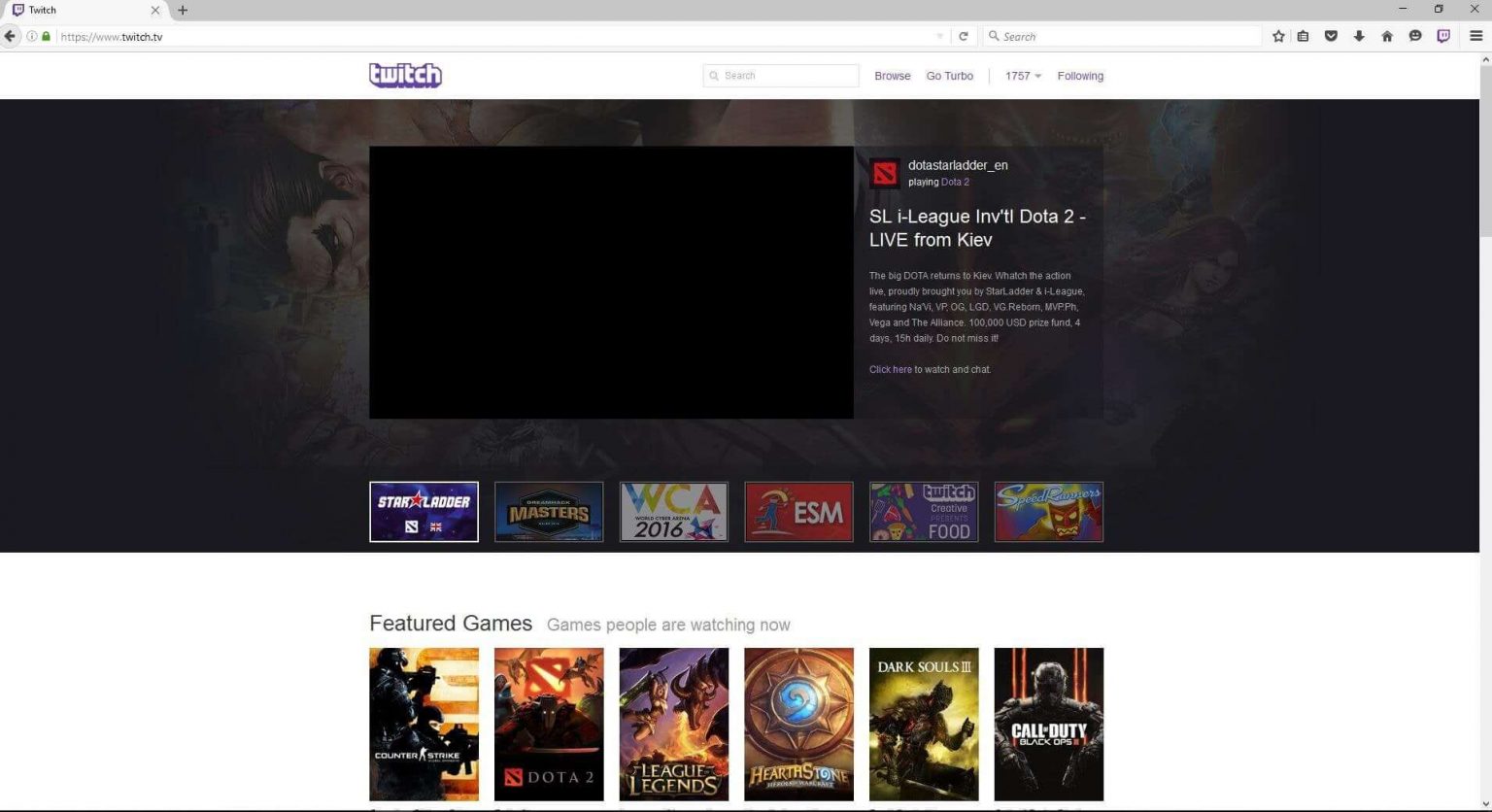Screenshot of the Twitch website displayed on a desktop or laptop browser, shown in a full browser window. The browser has a single tab open, labeled "Twitch" with the Twitch logo to its left. The URL bar confirms the site as "twitch.tv," and to its right are the browser's function icons, indicating the use of the Chrome web browser. 

The top section of the Twitch homepage features the Twitch logo in purple letters. Nearby, there is a search box alongside navigation links labeled "Browse," "On Turbo," "1957," and "Following." 

Central to the screenshot is a video player with no active video or audio displayed. To the right of the player, text reads "SL iLeague International DOTA 2, live from Kiev." The background of this section incorporates a dark, ominous DOTA-style logo featuring game characters. 

Below, the screenshot includes various game thumbnails, including "DOTA 2," "League of Legends," "Call of Duty," and "Dark Souls," along with links to other Twitch sections, such as "WCA 2016," "ESM," and "Star Loader," though these are small and somewhat difficult to read.